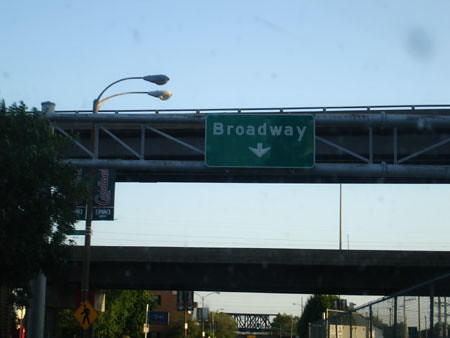This photograph depicts an urban scene captured from street level, focusing on the underside of a thick, multi-layered bridge structure. Dominating the foreground is a green highway sign with white letters that reads "Broadway" and features a downward arrow, indicating the road continues ahead. Attached to the bridge's edge, the sign stands out against the background. Alongside the bridge, a tall, white lamppost with bifurcated, curved lights extends over the road, and nearby, an additional pedestrian crossing sign in orange and a yellow diamond-shaped walkway warning sign are visible. The view hints at an intricate network of city infrastructure with yet another bridge visible in the mid-ground and a more robust, criss-cross trussed bridge in the distant background, possibly designed for heavier traffic like trains. A large chain-link fence runs down the right side of the road, enhancing the sense of an enclosed urban environment. The sky above is a clear, sunny blue, suggesting the photo was taken during the day, and the scene is bathed in a mix of light and shadow, subtly hinting at the approach of sunset.